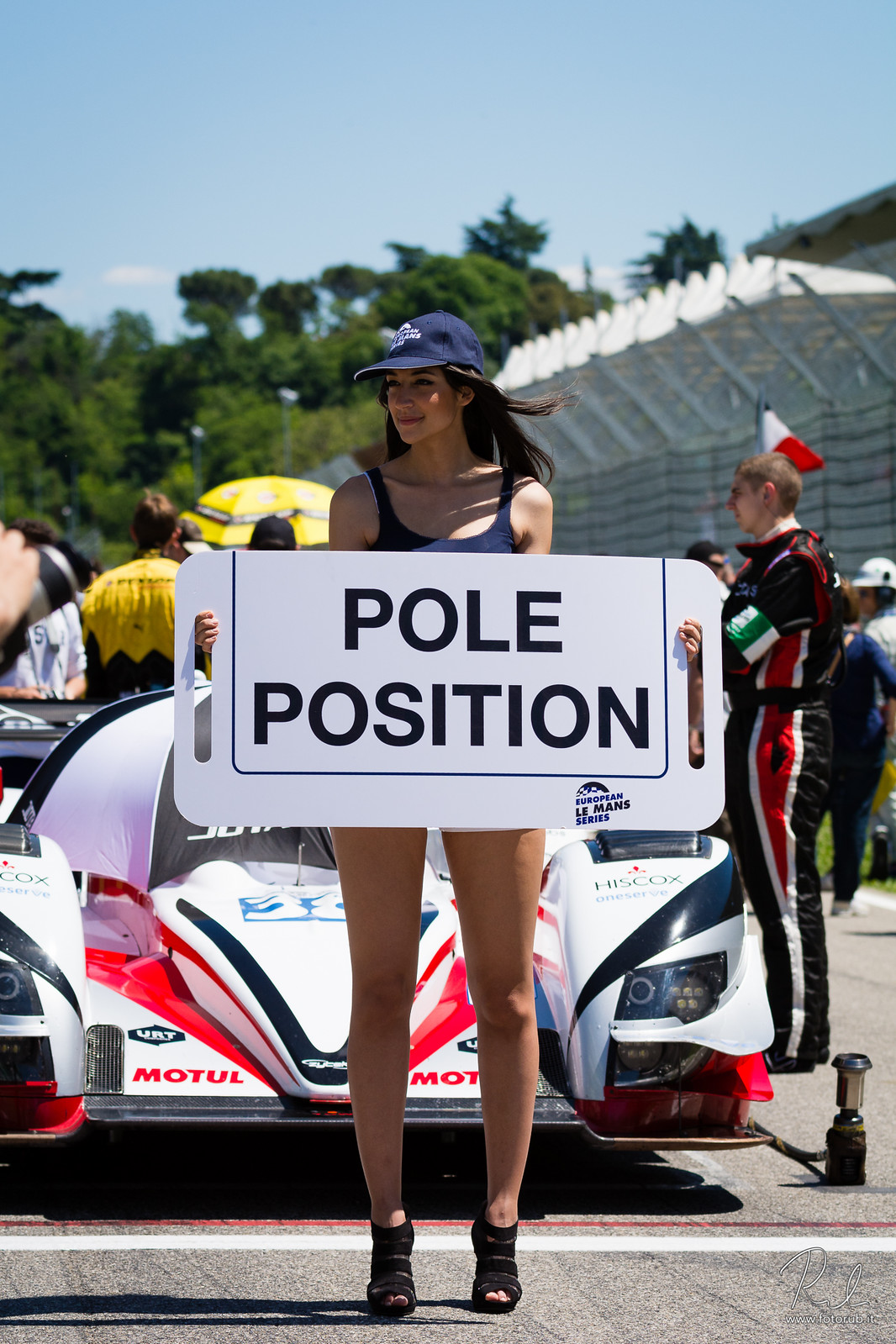In this vibrant photograph taken at a racetrack, a striking woman stands at the forefront, holding up a white sign with black sans serif lettering that reads "Pole Position." She has long, dark brown hair cascading from under a navy blue baseball cap adorned with a white logo. Complementing her cap, she's dressed in a dark blue tank top and black heeled sandals. While the lower half of her outfit is obscured by the sign, it hints at a short skirt or shorts. 

Behind her, a sleek white race car branded with MOTUL and other sponsors, featuring red and black stripes, awaits the race. The car is positioned against a backdrop of tall green trees and a vivid blue sky. Nearby, a race car driver in a black suit with red and white trim stands ready. Additional race crew members and another person in a yellow and black uniform can be seen, with vibrant details like a yellow umbrella adding to the scene's dynamic composition. The white stadium walls peek through in the background, framing this electric moment of anticipation before the race.